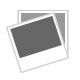This image features the trunks of what resembles roller skates or skateboard parts, presented as two identical sets of metal footplates and axles with wheels, one positioned slightly above the other. The silver footplates, crafted from shiny steel, are foot-shaped and exhibit a series of drilled holes along their sides. The wheels, four in total on each footplate, are thick with thin grooves, smooth, circular, and appear brand new, with a cream or light beige color. The lower set of wheels is fixed to an exposed metal footplate, while the upper set obscures part of the footplate underneath. Positioned on a tan background that casts light shadows, the footplates and wheels are meticulously clean, with the empty screw holes indicating the parts have never been used.